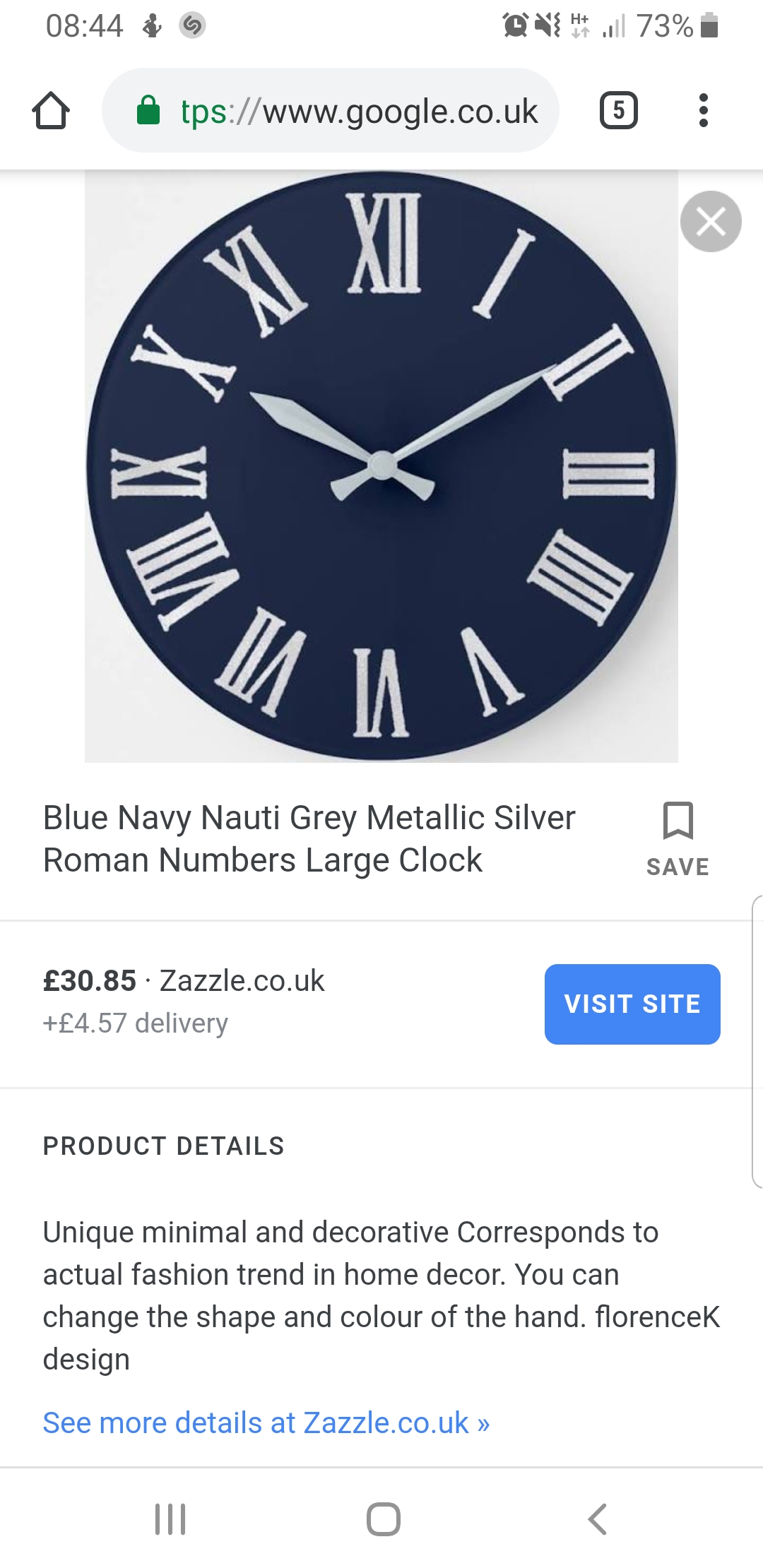This is a screenshot of a mobile phone displaying a Google search page. The web address shown is Google.co.uk. The search query appears to be about purchasing a clock. Below the search bar, there is an image of a clock. Detailed in the description beneath the image, the clock is characterized by a navy blue, metallic silver, and gray color scheme. It features large Roman numerals and is priced at £30.85. A blue button labeled "Visit Site" is visible, providing a link to the purchasing page.